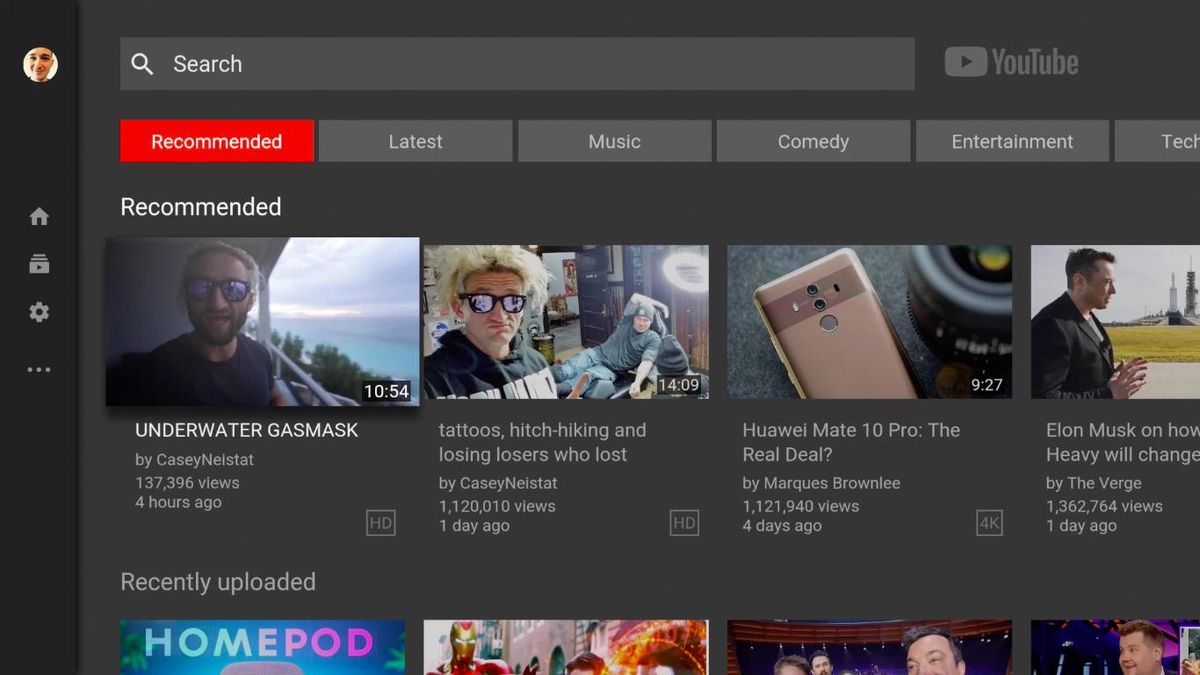The image portrays a predominantly gray, rectangular interface filled with a variety of text and data in different shapes and font types, forming various sentences. The content includes dates, numerical values, and specific times distributed across the interface. At the bottom, various clickable symbols indicate different functionalities. The top and right sides also feature distinct icons that grant users additional options. Scattered throughout the monochromatic background are blue hyperlinks, indicating interactive elements that can redirect users to other locations. Overall, the layout is designed for clear and concise data presentation, making it easy for users to absorb the wealth of information displayed.